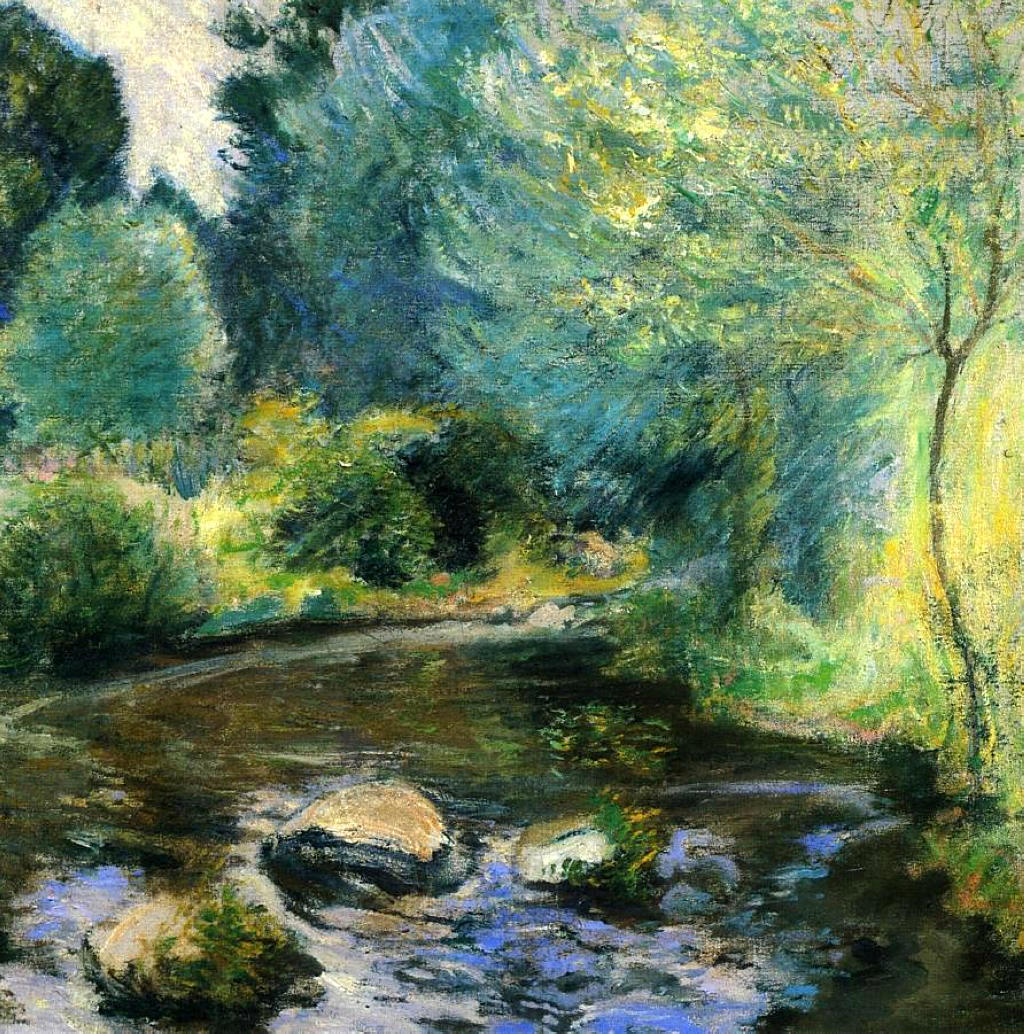This tall, rectangular painting, reminiscent of Monet’s style, depicts a serene forest stream, rendered in chalk pastel or rough color pencil. The bottom half features a dark, greenish creek dotted with smooth, dark gray boulders, some with green moss. The water, suggesting the movement of rushing water, converges towards the middle of the canvas before curving to the right. On the water's edges are various shades of green bushes and small trees. On the right side, a thin tree adorned with light green and yellow leaves, almost appearing aflame under the light, extends upwards. The left background showcases a light gray rock surface framed by dark green trees, with a hint of white sky in the top left corner. The artwork uses a palette of white, dark green, light green, yellow, brown, and black, with loose, implied strokes that reveal parts of the background paper. Measuring 8 inches wide by 8 inches tall, the composition contains no signature or date.